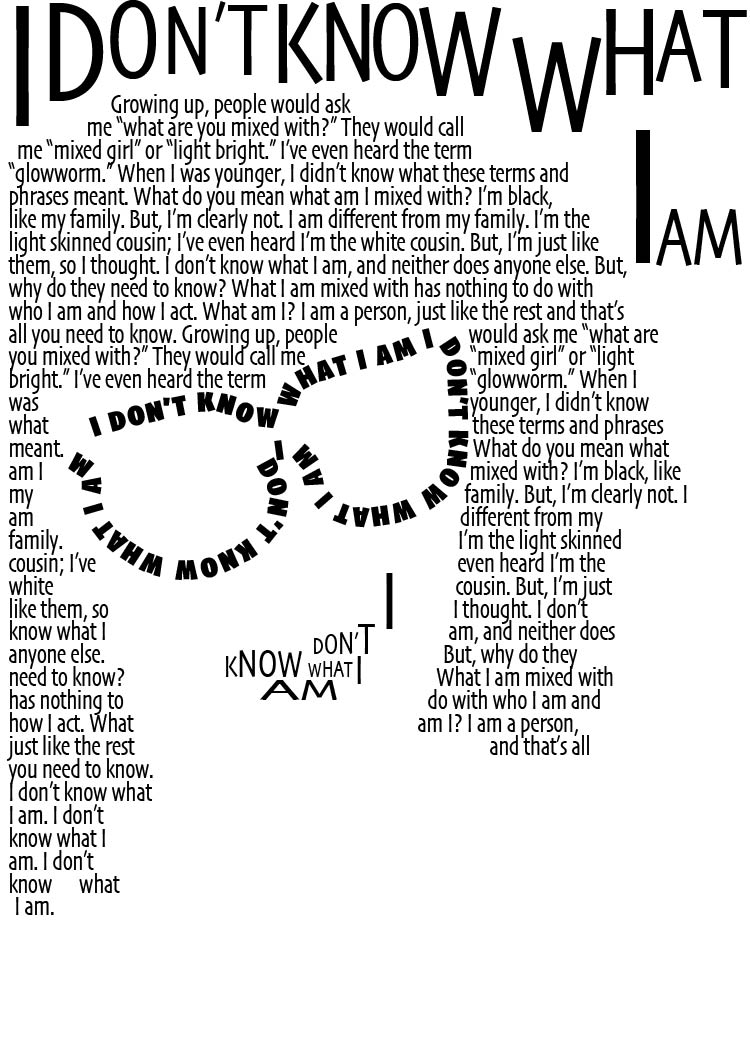This tall, rectangular piece of word art features a profound narrative set against a completely white background. Dominating the top in a bold font, the phrase "I don't know what I am" introduces the theme. Below it, a long paragraph traces the shape of a face adorned with glasses, with the glasses and mouth also formed by the repeated phrase "I don't know what I am." The narrative explores the deeply personal experience of growing up as a mixed-race individual, touching on the identity struggles and societal labels encountered along the way. Terms like "mixed girl," "light bright," and "glow worm" underscore the confusion and otherness felt. The text delves into the internal conflict of being part of a Black family while distinctively appearing different, often referred to as the "light-skinned cousin" or even the "white cousin." Ultimately, the paragraph asserts that what one is mixed with shouldn't define who they are or how they act, emphasizing their humanity and individuality: "What am I? I am a person just like the rest. And that's all you need to know." This repeating message continues along the left and right sides, creating the appearance of hair, rounding out this intricate and thought-provoking artwork.